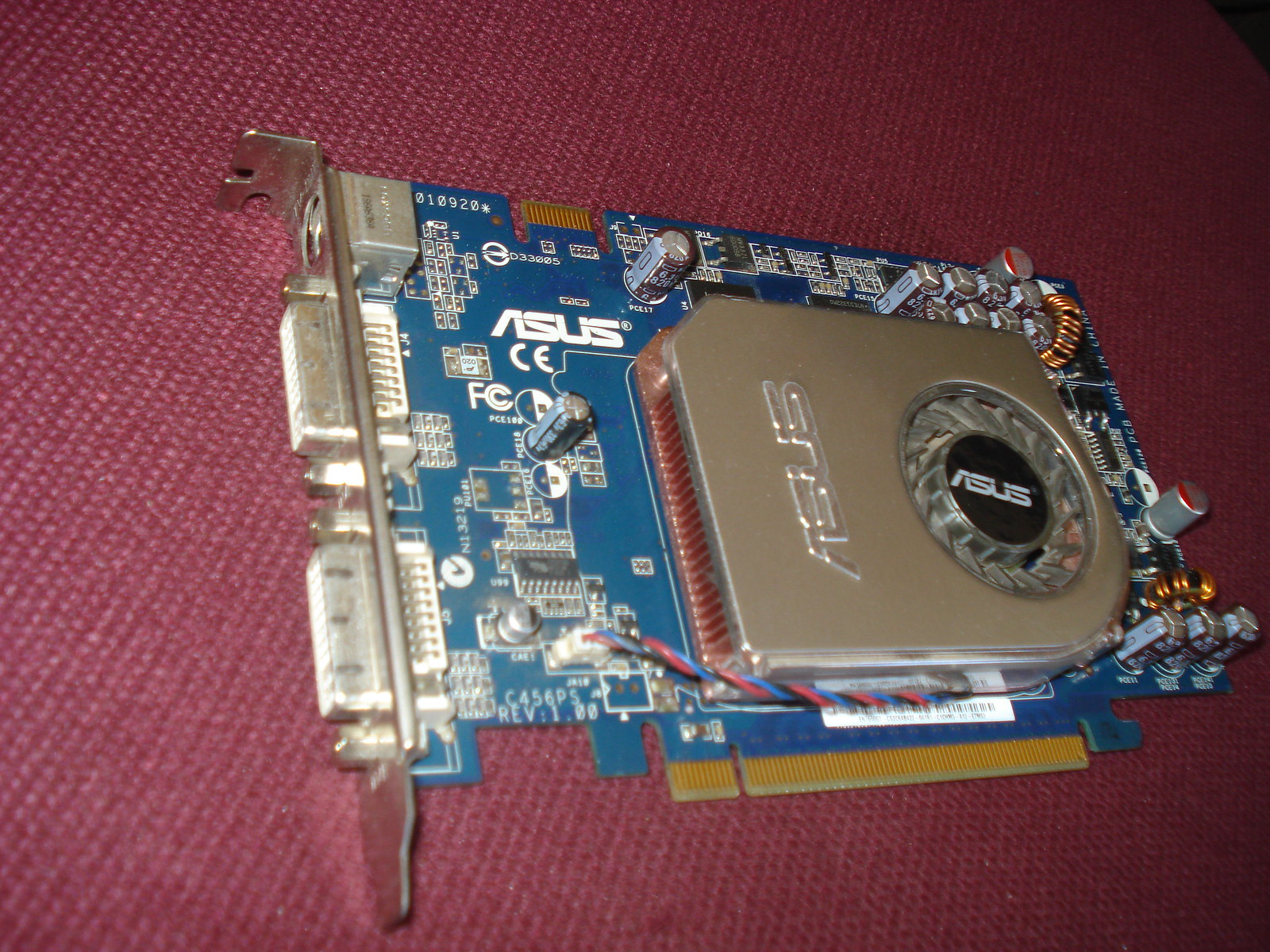This photo features an older-style ASUS graphics card displayed against a maroon, netted material that resembles a tablecloth or cushion. The graphics card is compact, suitable for a PCI slot, and predominantly blue. The cooling section boasts a single fan with "Asus" prominently displayed in raised letters on the casing as well as printed on the fan itself. "Asus" is also visible on the circuit board. Near the bottom of the card, the model identifier "C456PS Rev 1.00" is inscribed, although the exact model remains indiscernible due to a blurry white sticker beneath the cooling area. This card's vintage nature is highlighted by its solitary cooling fan and smaller size compared to contemporary graphics cards.